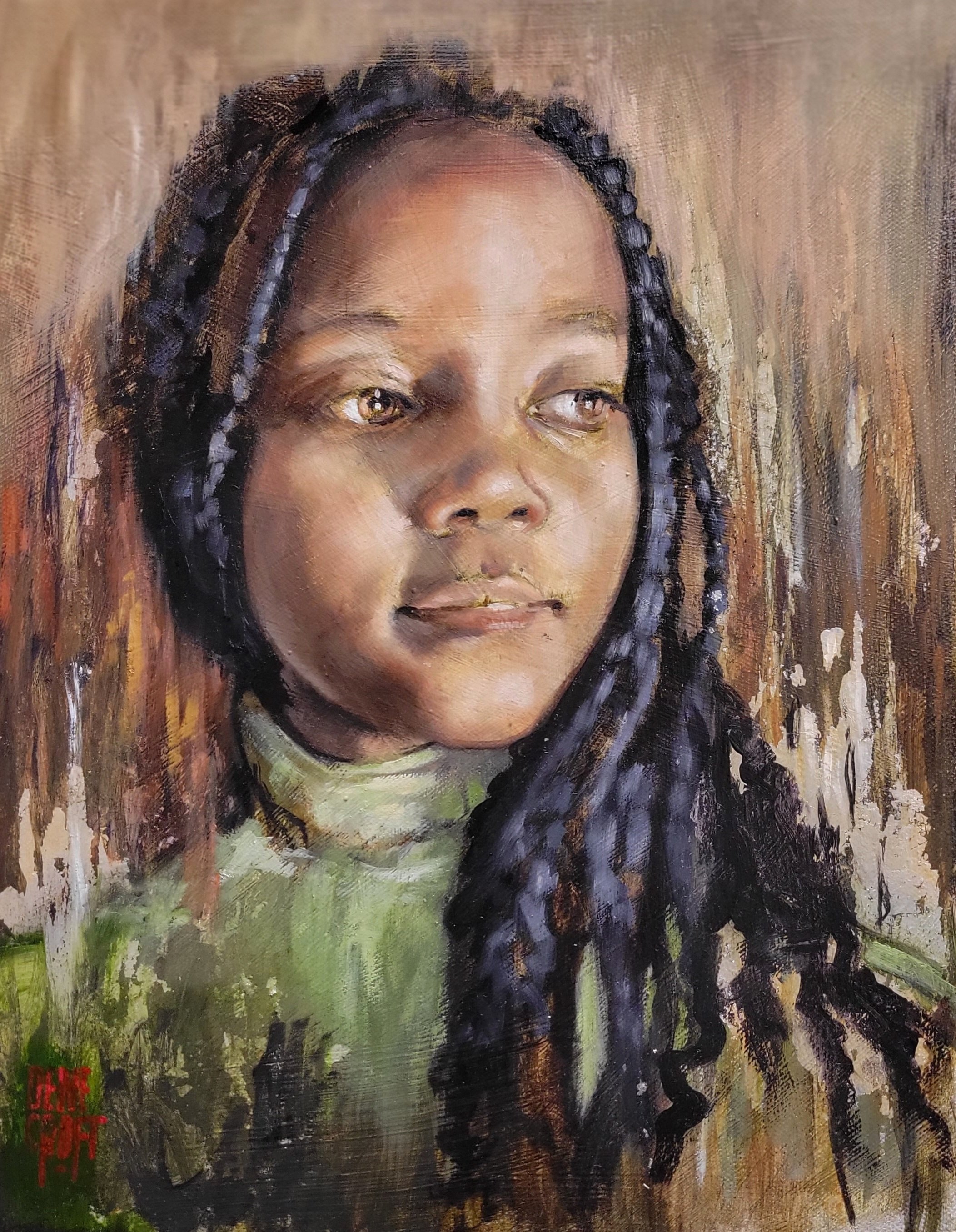The painting captures a young African-American girl with long, intricately braided hair, some braids cascading over her left shoulder while others tuck behind her head. Her gaze is directed towards the right, giving her a contemplative and somewhat melancholic expression, enhanced by lifelike detailing in her eyes and nose. She appears to wear a green turtleneck sweater, masterfully rendered with layers of paint that create an ombre effect and feature streaks of orange, red, light green, and dark green. Her shirt also sports a vibrant pop of red and some brown or golden hues. The background imitates the texture of wood, with vertical brown, white, and yellowish streaks, further enriching the painting's depth. Her face stands out as particularly realistic, with a prominent forehead, bold yet moderately sized lips in a half-smile, and eyes that resonate with emotions. The intricate use of paint highlights not just her physical features but also an underlying emotional narrative.